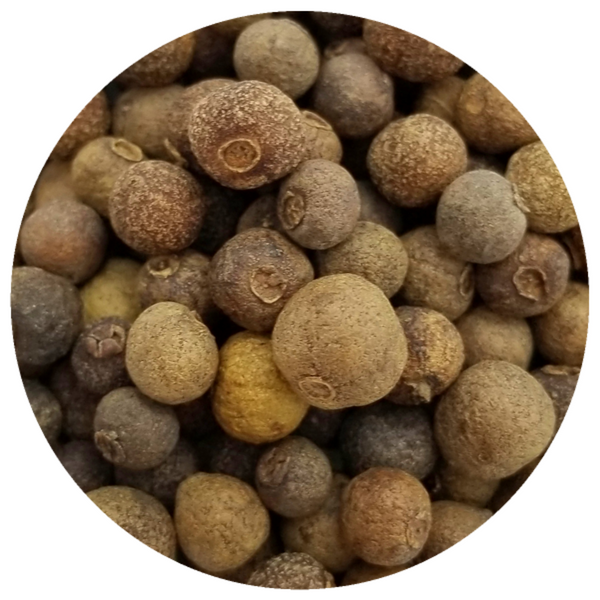This circular-cropped image, set against a white vignette background, captures a multitude of organic round seeds or nuts, each approximately the size of a blueberry. The main subjects vary in color, ranging from dark chocolate brown to shades of beige and yellow, with some displaying tan and even darker reddish hues. These seeds are densely piled together, totaling nearly a hundred. Each seed features a small circular mark or pit, indicative of a natural opening or where it was once attached to a stem, suggesting they might be dried or roasted. The detailed texture and color variations create an intricate and visually appealing composition.